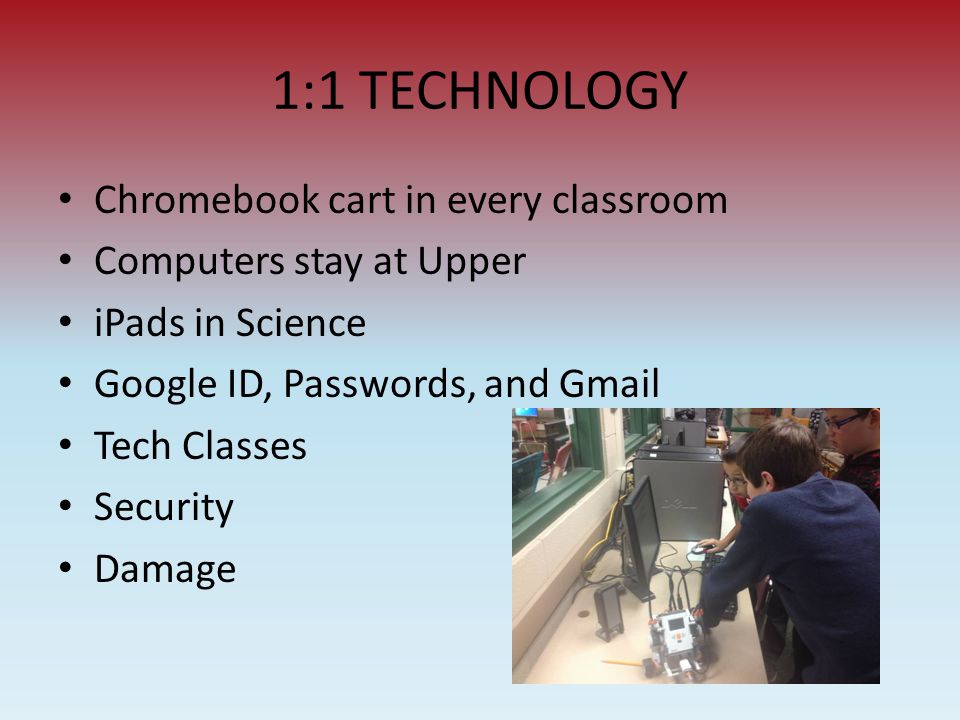The PowerPoint slide features a gradient background transitioning from dark red at the top to lighter blue at the bottom. The title of the slide, "1-to-1 Technology," is prominently centered at the top in black text. Below the title are seven bullet points, each in black text, detailing the key components: "Chromebook cart in every classroom," "Computers stay at upper," "iPads in science," "Google ID, passwords, and Gmail," "Tech classes," "Security," and "Damage." In the bottom right corner of the slide, there is a photograph depicting three young boys, likely around eight to ten years old, gathered around a computer setup that includes a monitor, keyboard, mouse, speakers, and a homemade robot connected with cords and wires. The boys, two of whom are wearing glasses, are engaged in what appears to be a classroom or laboratory environment.